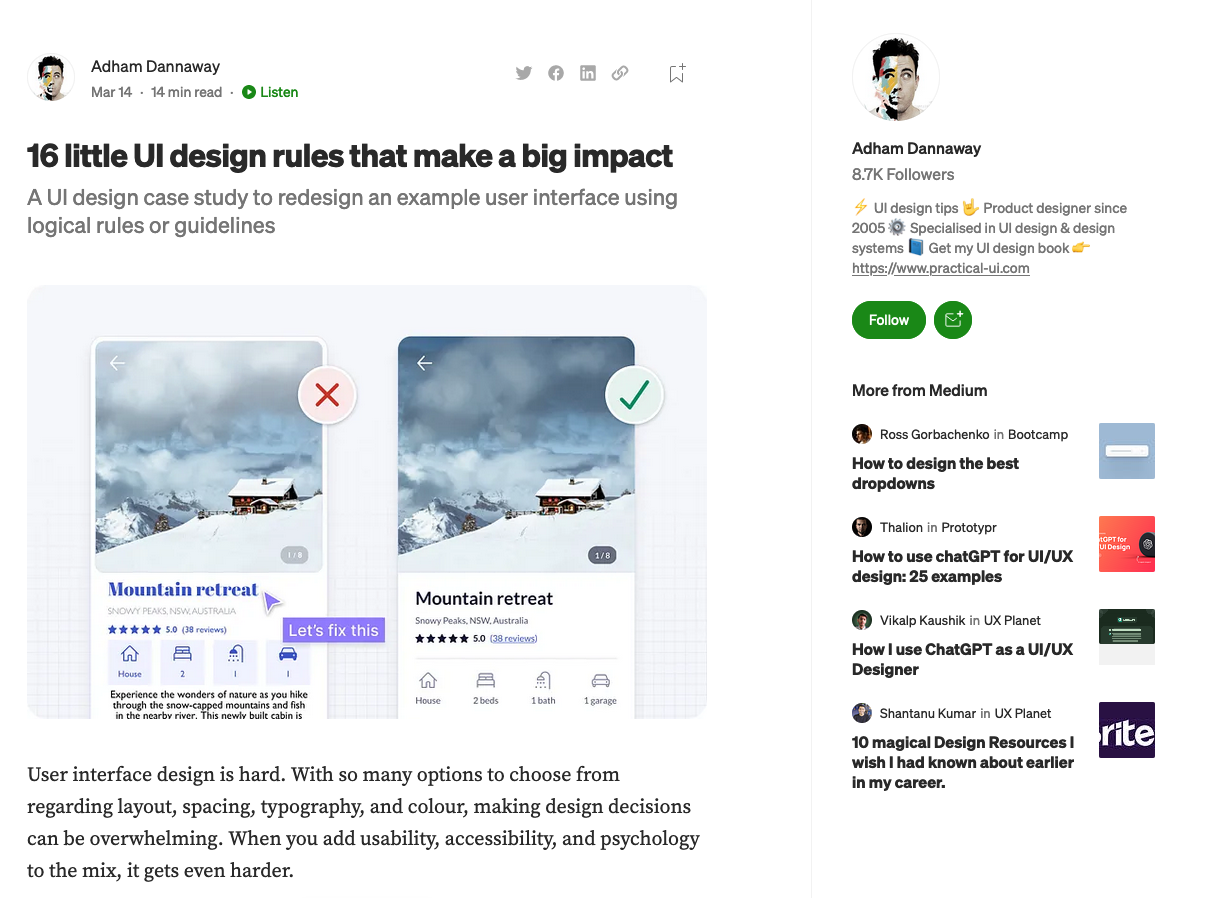In the image, there is a snapshot of a web page header that features content related to UI (User Interface) design. At the top, it displays the user's handle, "addhimDannaway," spelled as "a d h i m d a n n a w a y". Below this, it mentions the date "March 14" and specifies that the article is a "14 minute read." There is also an option to listen to the article with a "Listen" button.

The headline of the article reads, "16 Little UI Design Rules that Make a Big Impact." Below the headline, there is a subheading describing the article as a "UI design case study to redeem an example user interface using logical rules or guidelines."

Within the image, there is a background picture of a mountain retreat that initially shows white clouds with a bit of gray. This background changes to display darker clouds with some white. The revised design with darker clouds is marked with a green checkmark indicating correctness, while the original design with whiter clouds is marked with an "X" in a box, suggesting it was incorrect.

Additionally, the text elaborates on the challenging nature of UI design by highlighting the various factors a designer must consider, such as layout, spacing, typography, and color. It emphasizes that making design decisions can be overwhelming, especially when usability, accessibility, and psychology are also factored in.

On the side, there is a section where readers can choose to follow the author and read more of his content.